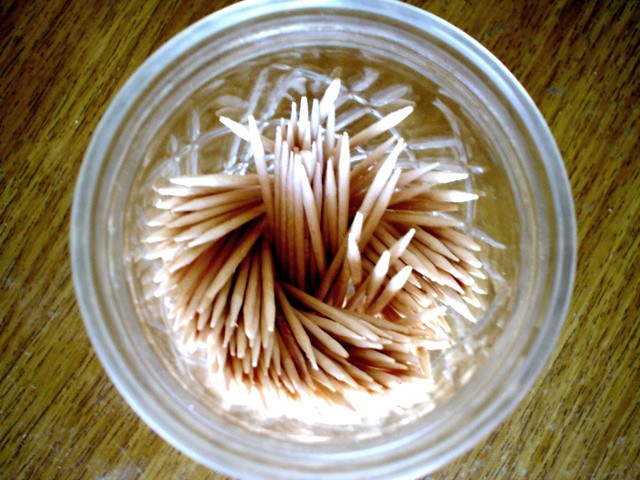The image captures an overhead view of a clear glass container filled with numerous toothpicks, estimated to be between 50 to 100 in number. The toothpicks, thick and irregular, are arranged in a somewhat spiral formation, resembling a flower shape, with some pointing in different directions and others standing upright, forming a counterclockwise circular pattern. The glass, which features a distinguishing lip and crystal-like markings on its sides, rests atop a wooden surface with a light brown and black grain running diagonally across the frame. The scene is illuminated by a mix of yellowish indoor light and natural sunlight, which causes some of the toothpicks to appear brightly lit and slightly overexposed, especially towards the center, creating shadows and variations in clarity. The overall composition has no people or text, focusing solely on the intriguing arrangement of toothpicks in the glass on the wood-grain table.